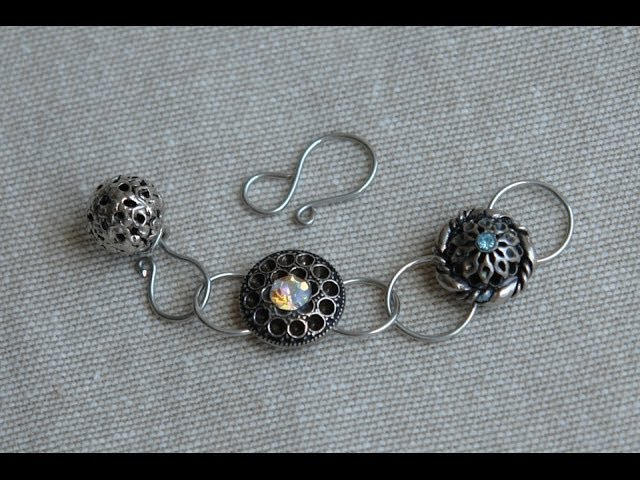This detailed close-up image features three interconnected pieces of silver jewelry, all laid out on a gray, carpet-like background. The primary piece appears to be a small, round, hollow bell about the size of a pea with a loop on one end, which is hooked onto a larger circular silver ornament. This larger ornament has a smooth metal surface with two loops at either end, allowing it to be connected to both the bell and another similar circular ornament. Each connection is facilitated by silver rings. Additionally, there is a singular metal hook lying above these interconnected pieces, which seems designed to potentially close the loop by attaching to one of the pieces below. Throughout the jewelry, there are intricate details, including one piece that features a blue stone and another that has a tiny picture embedded within.